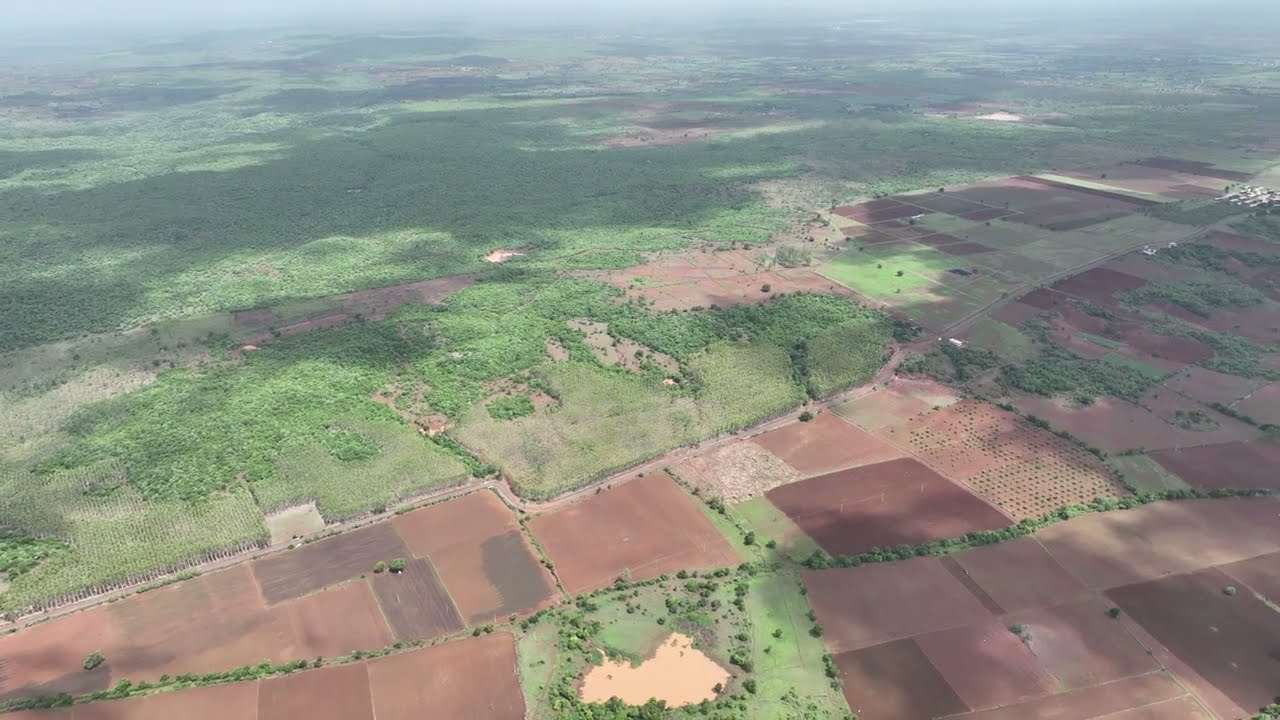This aerial photograph, likely taken from an airplane or drone, presents a high-altitude view of a vast and mostly flat landscape, dominated by a patchwork of agricultural fields. From this elevated perspective, the land below is categorized into clear, parceled-out rectangles and squares, primarily seen in the foreground and the lower right portion of the image. These fields exhibit shades of brown and tan, indicative of plowed earth or sandy soil. Centrally, a sandpit is noticeable, encircled by greenery and a line of trees, possibly serving as windbreaks. 

In contrast to the organized farmland, the upper sections of the photograph, particularly towards the left, showcase lush, green vegetation that appears more natural and untamed, likely comprising pastures, thick grass, bushes, or even dense tree canopies, though it's hard to distinguish individual elements from this height. Sparse roads can be spotted weaving through the landscape, yet no clear residential structures are evident, suggesting a predominantly rural, agricultural area. However, a long structure and a series of smaller buildings are faintly visible on the far right, potentially indicating some form of habitation or farming infrastructure. The overall scene is under a hazy sky, contributing to a serene and somewhat ambiguous summer atmosphere.